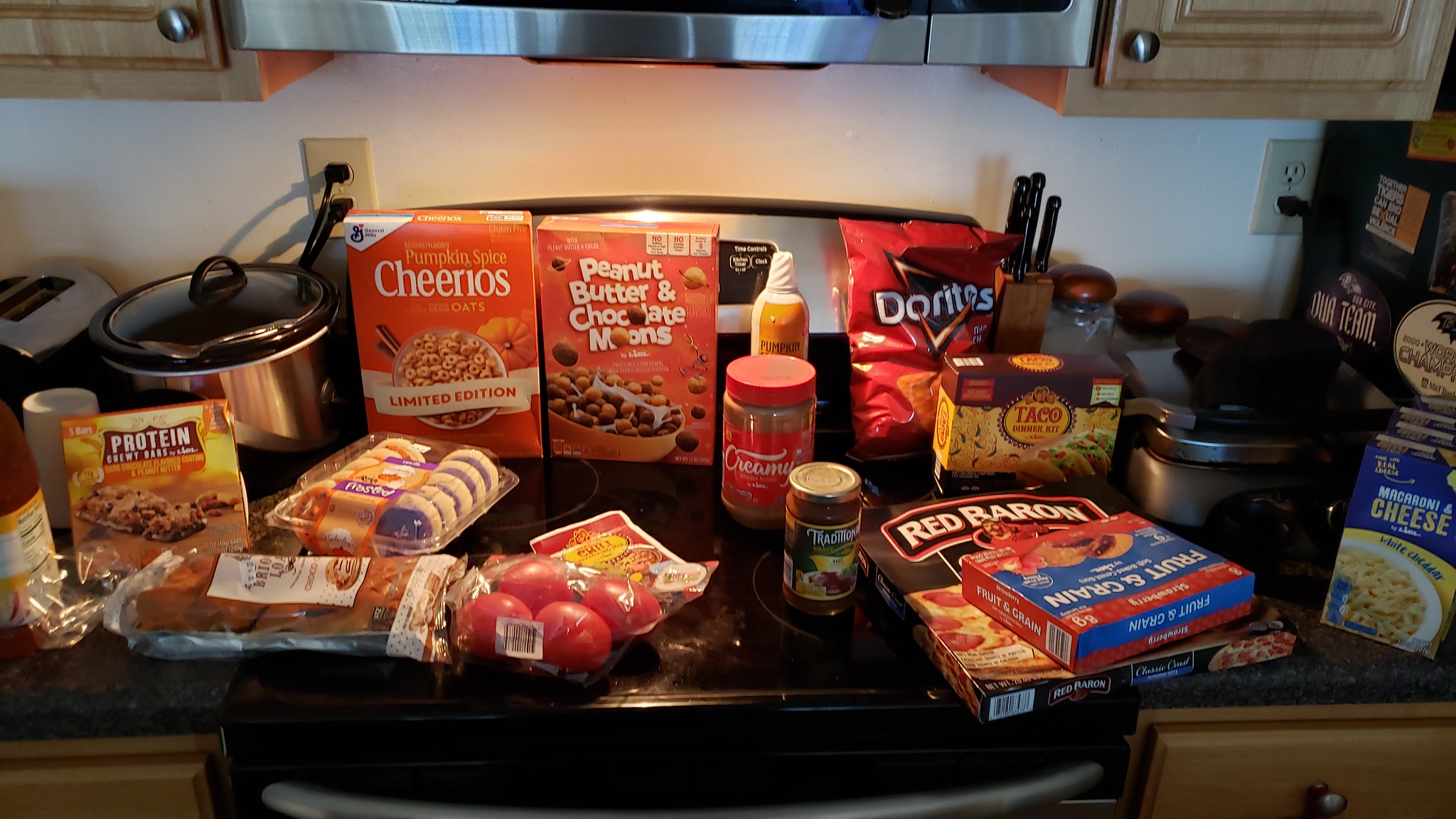A meticulously organized kitchen scene unfolds in the image. At the top left, a sleek cabinet with a silver handle and metal strip across its center stands out. Adjacent to it is another matching cabinet, separated by a pristine white wall. Below the left cabinet, a misplaced white sock lies with two bugs nearby. Centralized in the scene, another cabinet features a silver upper section and a black lower section. Both the left and right cabinets are finished in a rich brown, adding warmth to the composition.

The main focus of the scene is a plethora of grocery items scattered across the countertop. Among the assortment, a Red Baron frozen pizza box is prominently displayed. To its side, two cereal boxes brandish the Cheerios label, one variety being peanut butter and chocolate-flavored. A bag of Doritos and a taco seasoning packet suggest an impending festive meal. Nearby, a cheese box rests next to a pack of fresh tomatoes encased in plastic. A pack of cookies and a Wiggles-branded item adds a touch of indulgence to the mix. Further to the right, an ice cream carton sits atop a kitchen block, promising a sweet finish.